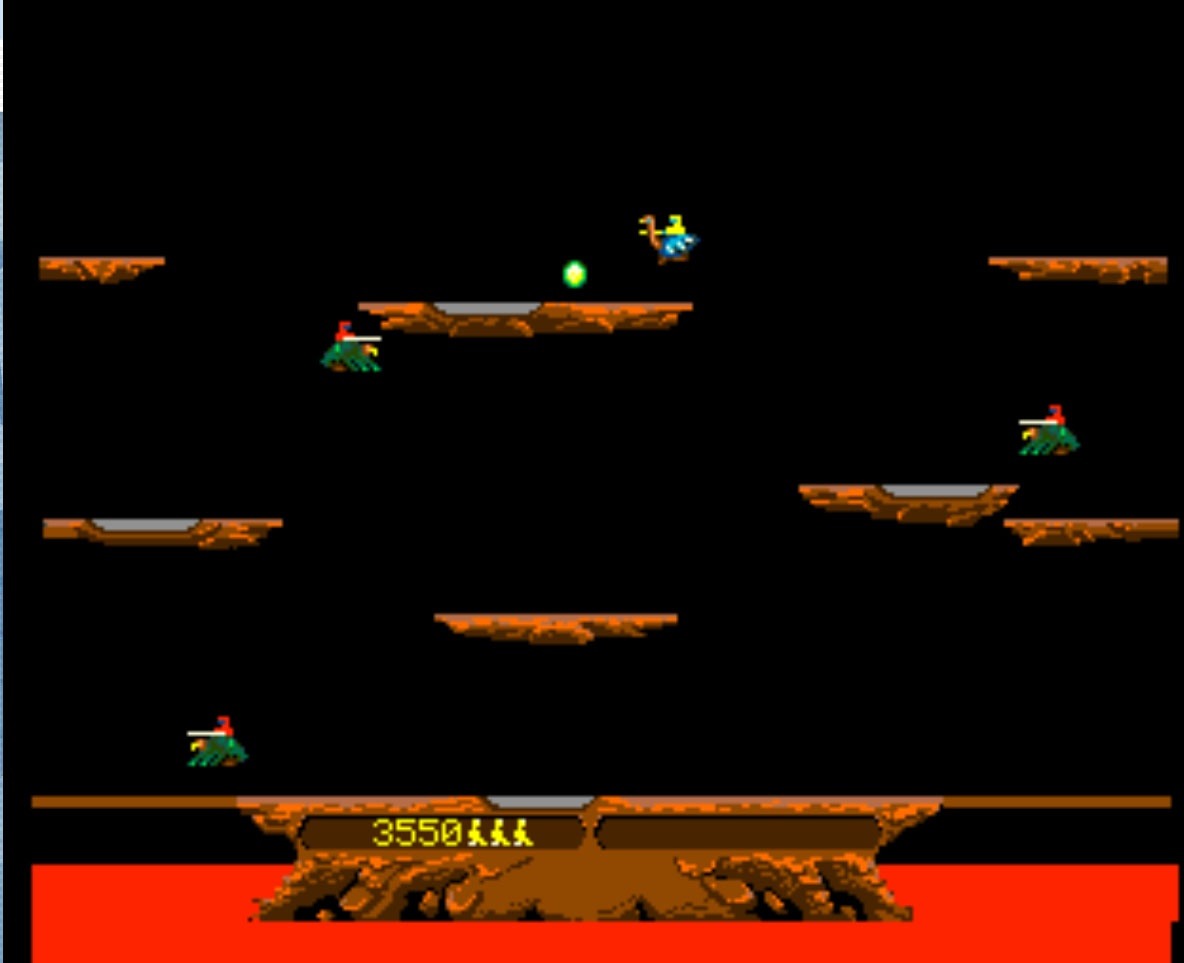This screen capture from an unidentified video game features a stark black background. In the bottom left corner, a score of 3550 is prominently displayed, with an area on the right seemingly reserved for a second player's score, which remains empty. Along the bottom edge of the screen runs a large red stripe, accentuating the interface. The gameplay area consists of approximately seven or eight shelves of varying heights, populating the screen vertically. Different animals animate these shelves, with one in particular appearing to be under the player's control. It is uncertain whether the player controls an animal or a ball, but it seems the goal is either to navigate the animal to catch the ball or to maneuver the ball to hit the animal, as both move from shelf to shelf in this challenging and dynamic environment.